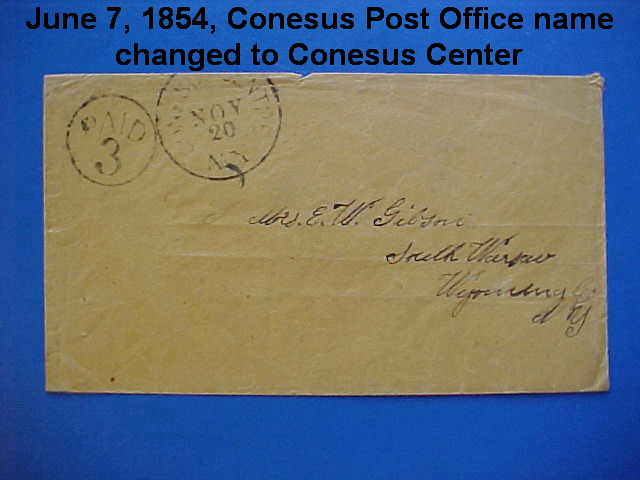The image shows a very old, discolored brown envelope, which appears to have originally been white, but has since faded to a yellowish dark color. The envelope is displayed on a blue background, on which is printed in black font, "June 7, 1854, Conesus Post Office, name changed to Conesus Center." On the envelope, there are two notable stamps: one circular stamp marked "Paid 3" and another that reads "November 20," suggesting a postmark. Handwritten in black ink towards the center of the envelope is the recipient's address, intended for a "Mrs. E. W. Gibson." Though the full details are unclear, it mentions South Wyoming. The details date the letter to the mid-1850s and imply it originated from Conesus, New York.